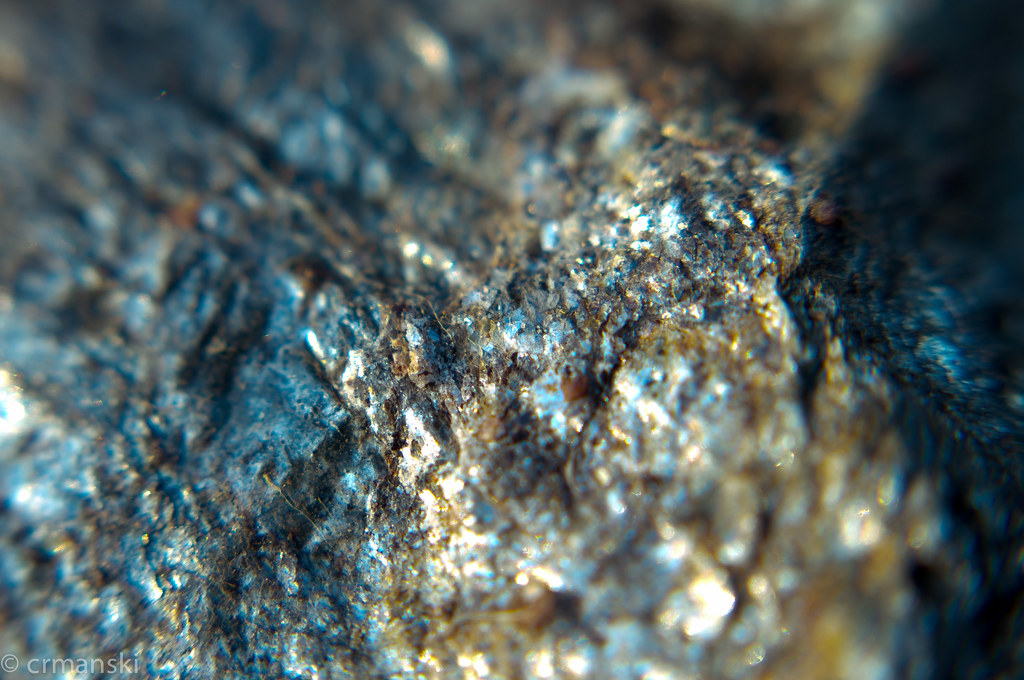The image is a large, horizontally aligned rectangular photograph of a stone that appears to be pyrite. The photograph lacks borders and is predominantly blurry, except for a clearer area in the center. The stone is primarily dark with accents of gold, brown, and white. The focused central section reveals additional colors, including blue, maroon, and gray, with shiny white specks. The stone has a variety of textures, with smoother areas in the upper right and rougher areas in the lower left. In the lower left corner, the image bears a copyright symbol followed by the name "C. R. Manske" in white lowercase letters.